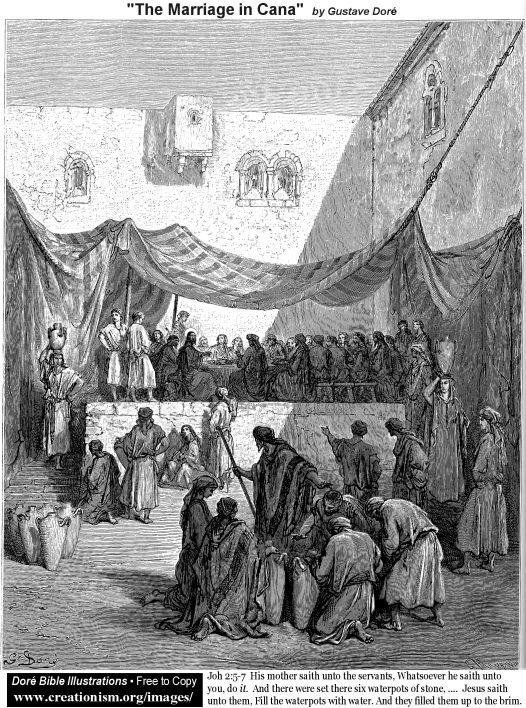The black-and-white image appears to be a meticulously detailed, hand-drawn illustration, likely created with pencil by the artist Gustav Doré, and is titled "The Marriage in Cana" as indicated in bold at the top. This biblical illustration, free to copy and sourced from www.creationism.org/images, captures a significant moment described in the Book of John 2:5-7, where Jesus performs the miracle of turning water into wine at a wedding feast. 

The scene is set in an ancient Middle Eastern context, evidenced by the architectural features in the background, including a white brick building with a few windows. Central to the composition is a large cloth tent, propped up with stakes, creating a canopy under which a considerable crowd of about fifty people has gathered. Many of these figures are donned in robes, clearly situating the tableau in historic times. At one end of the table beneath the tent, a woman is depicted carrying a vase on her head—a common practice for transporting water. 

In the foreground, a man with a staff, possibly a shepherd, is a focal point, drawing the attention of onlookers, some of whom are kneeling, perhaps in prayer or reverence. The illustration also shows people seated on a stage, which has steps leading up to it, engaging in the ceremonial activities of the feast. Each character in the gathering is portrayed in intricate detail, emphasizing the artist's skill in capturing the essence of the historical and spiritual significance of the event. The quote inscribed at the bottom right, “His mother saith unto the servants, ‘Whatever he saith unto you, do it.’ And there were set there six waterpots of stone. Jesus saith unto them, ‘Fill the waterpots with water,’ and they filled them up to the brim,” further highlights the miraculous event being depicted.